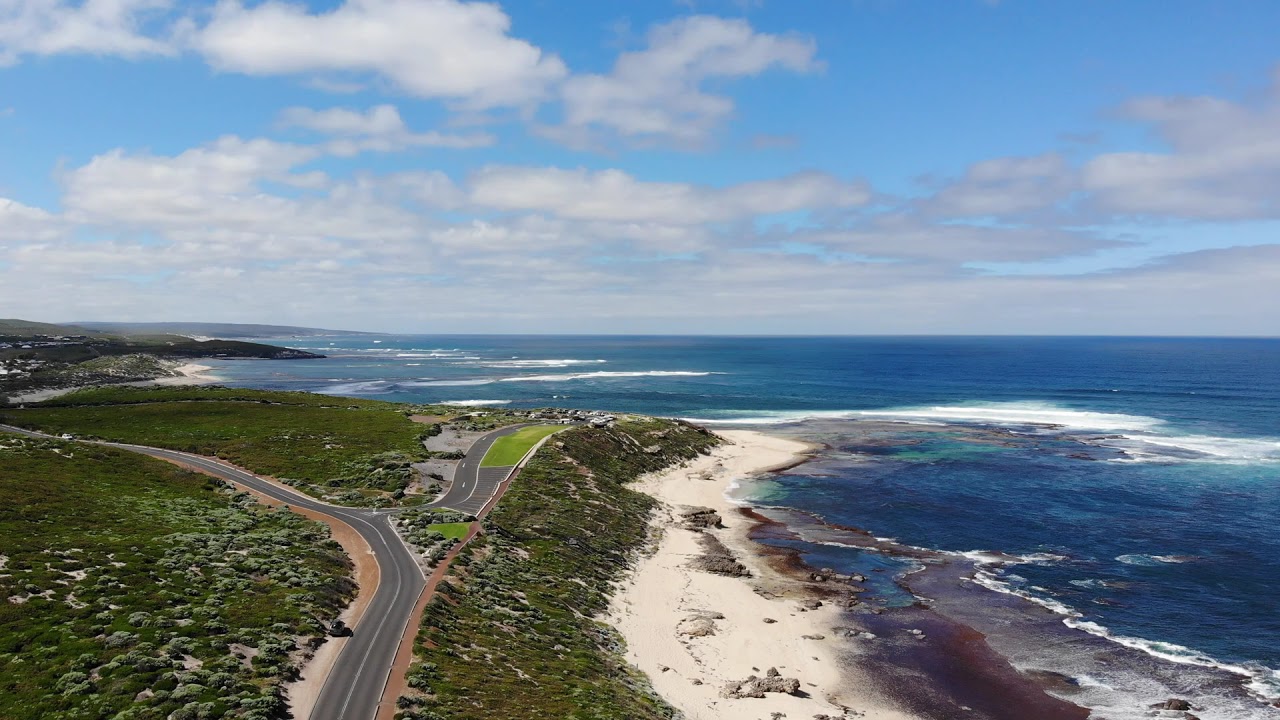The image is a bright and clear aerial photograph taken during the daytime, capturing a coastal scene from above. Dominating the right side of the composition is a vast, dark blue ocean with waves gently crashing onto a sandy white beach, creating a gradient of sand colors from dark near the water to lighter hues further up the shore. The left portion of the image features a winding gray roadway, stretching from the bottom left corner into the distance, alongside lush green grass and bushes. A lone white vehicle is visible on this road, suggesting it provides access to the serene beach area. The overhead view reveals no buildings, emphasizing the natural landscape. The upper third of the image showcases a bright blue sky speckled with white, puffy clouds, enhancing the overall sense of tranquility and open space. The combination of natural elements and the clear, well-lit setting underscores the vivid and representational nature of this drone-captured photograph.